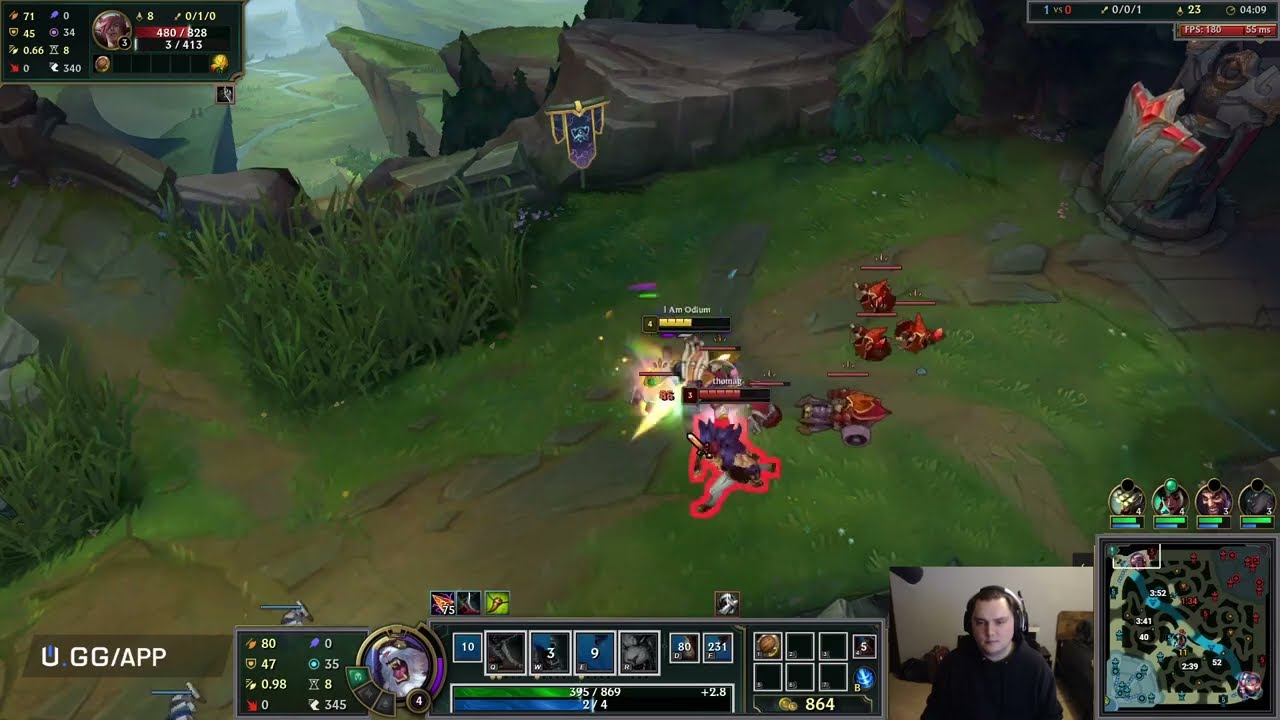This colorful screenshot from a video game, likely taken from a live stream, features a horizontally rectangular image without a border. In the bottom right corner, a real gamer is depicted in a small video overlay. The gamer, a young man with brown hair, is seated facing the viewer, wearing a dark long-sleeved shirt and a headset with an integrated microphone. Behind him, part of a microphone is visible, indicating he is in his room.

To the right of the gamer’s overlay, there's a square map showing the gaming field. To the left, another rectangular box displays numbers and figures, while the letters "UGG/APP" appear in the far left corner. At the top of the screen, a rectangular box presents additional numerical data.

The in-game environment showcases an outdoor scene with tall green grass, rocky pathways, and a small valley with a river running through it. Central to the image are several characters, one of whom appears to have been defeated, lying on the ground with a red outline around their body. Scattered around this character are various objects, possibly weapons. The setting, possibly resembling a forest, includes elements like stone and maybe even a dirt road leading deeper into the forest.